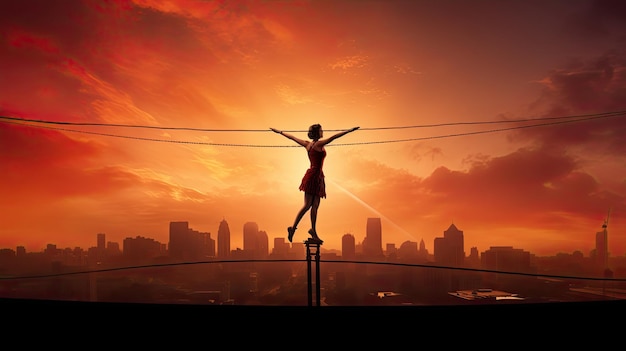In this fanciful and atmospheric image, a young woman, dressed in a red ballerina outfit that extends halfway down her thighs, is seen balancing gracefully on a thin black pillar that extends upward from a broad black bar at the bottom of the scene. Standing on one foot in a classical ballerina tippy-toe pose, she holds her arms extended horizontally, creating a striking silhouette against the vibrant backdrop. Her medium-length hair is styled into a bun, adding an elegant touch to her poised form as she gazes slightly upward and to the right.

The background is dominated by a dramatic sunset scene, where the sky transitions from a bright yellow burst at the sun’s center to various shades of orange and deep red, enveloped by a stretch of vivid clouds. Below this resplendent sky, the silhouetted skyline reveals a jagged array of tall and short buildings, casting an urban charm from the left to the right of the image. Dark silhouetted telephone wires add depth to the composition, running horizontally across and around the figure, enhancing the overall sense of height and balance in this captivating photograph, which evokes the feeling of an exquisite oil painting.